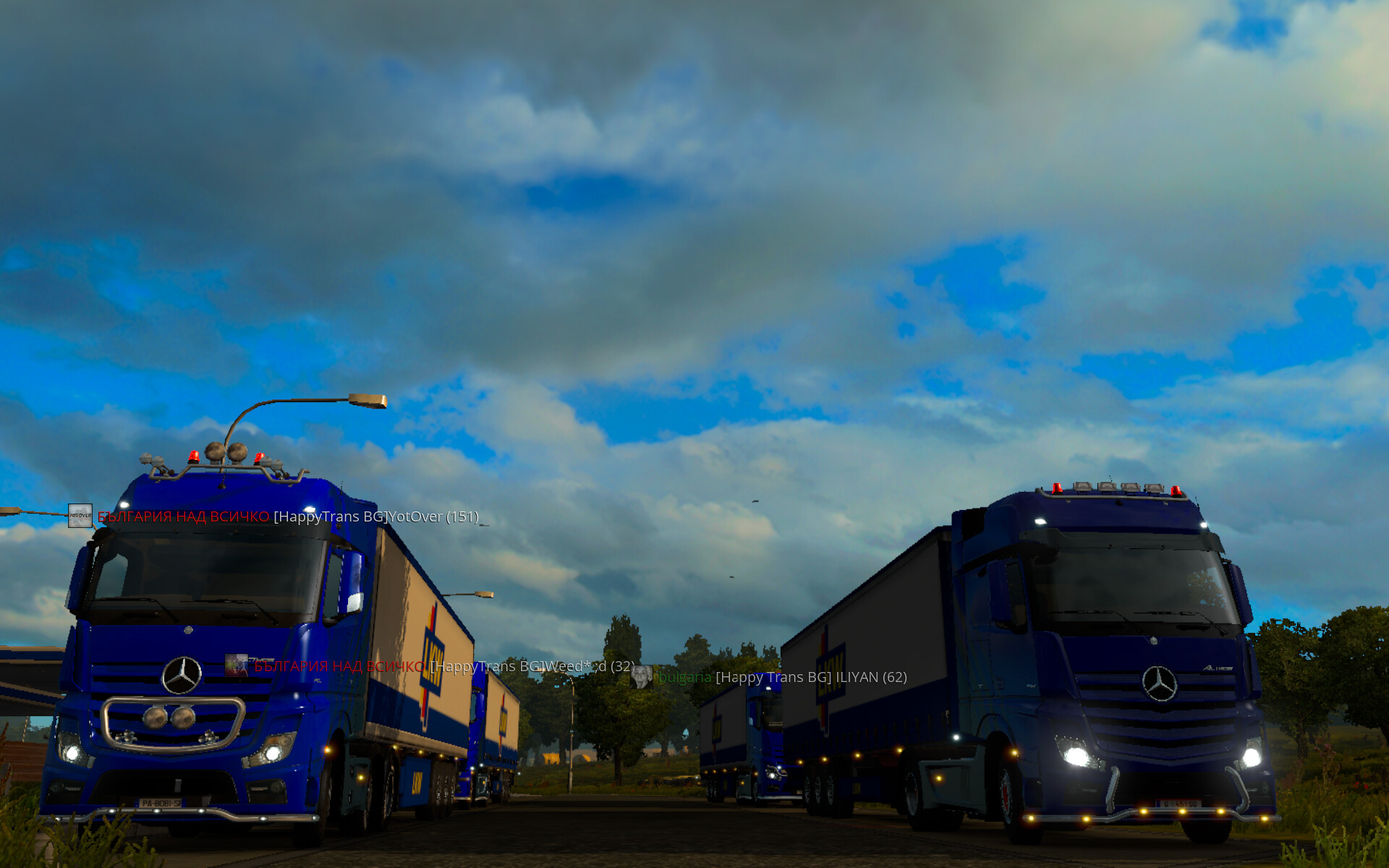A nighttime street-level photograph presents a scene framed between two parallel Mercedes cab-over-style tractor-trailers, positioned to the left and right. Both trucks feature blue cabs with their lights on, highlighting their distinct presence in the dark. The left truck is a double trailer with a cab-over design, decorated with temporary white boxes bearing an emblem. Emblazoned on the side are the letters "LKW" in white, alongside a color scheme of blue, white, and yellow. The right truck, also a Mercedes, pulls a single trailer under similarly dark conditions, providing limited detail due to the dim lighting.

Amid the darkness, the background reveals a sky under thick clouds with spots of blue peeking through. Distant trees stand silhouetted against the obscured sky, contributing to the eerie ambiance. The image, potentially AI-generated, includes textual elements in different languages and logos. Notable inscriptions like "Happy Trans BG," "YOT over 151," and "62 in parentheses" are subtly blended against the scene, likely indicating brand names or model specifics. Running lights illuminate parts of the trailers, and two streetlights cast a minimal glow on the left, enhancing the nocturnal setting.